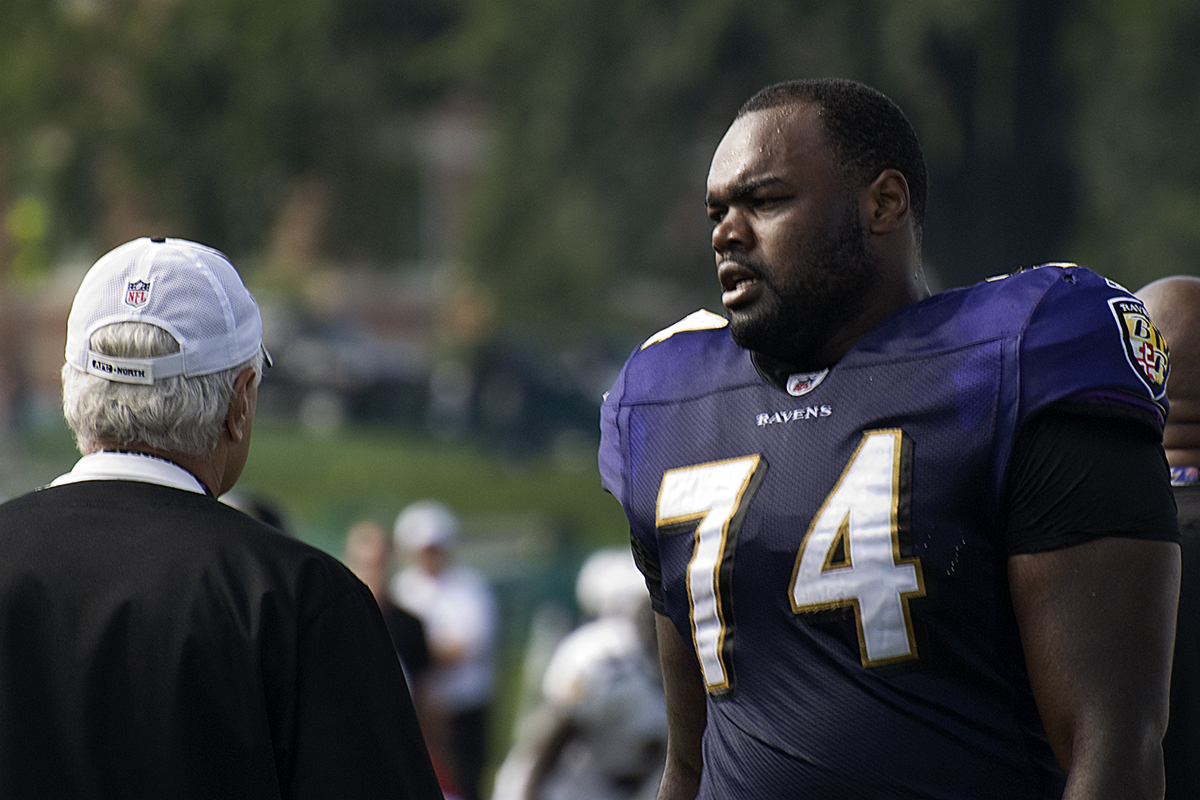The photograph captures a moment where a football player, donning a dark purple jersey with large white number 74 and the word "Ravens" near the neckline, engages in a conversation with an older man. The football player, who appears to be an African-American, dominates the right side of the image and is depicted with darker purple patches on his jersey from sweat. Notably, a SHIELD logo adorns his shoulder pad. The older man, significantly shorter and positioned in the bottom left corner, faces away from the camera, revealing only the back of his white baseball cap, which bears the NFL logo, and his black jacket over a white shirt. The player's open mouth indicates he is actively speaking. In the blurred background, various people, grass, and trees are faintly visible, grounding the scene in an outdoor setting. The photograph, rectangular in shape and horizontally aligned, captures this candid interaction vividly amidst a bustling, vegetative backdrop.